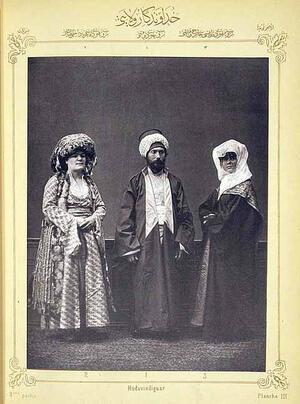The image features a black-and-white photograph encased in an aged, light brown frame with decorative designs at the top and corners. The frame also includes text in a foreign language at the top and a subtitle at the bottom, though the latter is blurry. The photograph shows three people standing and facing the camera, set against a dark grey background with a similarly colored floor. 

In the center is a man with a dark beard, dressed in dark robes that have a light-colored chest area, and wearing a large, turban-like headdress. To his left is a woman in a light-colored, striped dress with long sleeves, adorned with an additional piece of fabric tied around her waist and draping down the side. She also wears a large headdress that resembles a fabric cloth covering her hair. To the man’s right stands another woman, clad in a dark robe and wearing a light-colored fabric head wrap that covers her head and neck.